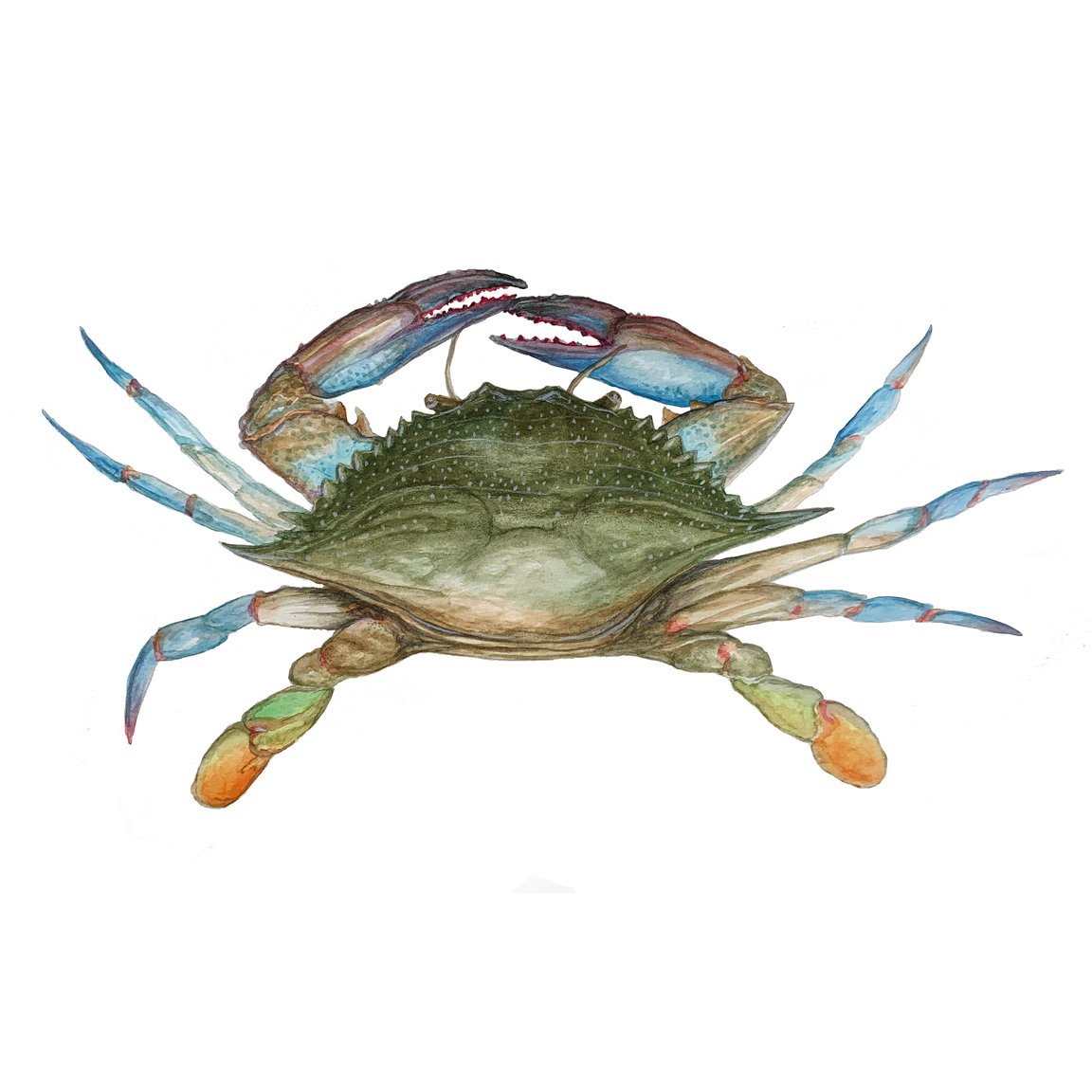The image is a highly detailed colored pencil and possibly watercolor illustration of a crab on a blank white background. The crab is depicted from a 45-degree top-down angle, presenting a lifelike and realistic appearance with complex shading and texturing. The crab's shell is primarily a dull green with sharp, jagged edges that form an oval shape with pointed sides. The eight legs exhibit varied hues; the rear legs are tipped with orange, transitioning to green, while the next three pairs on each side are brown towards the body and fade into light blue at the tips. The pincers are brown and blue with hints of red. The shell also contains blue and brown elements, adding to the depth and realism of the rendition. Despite its stylized and somewhat loose drawing style, the crab's vibrant yet earthy tones of green, blue, brown, and orange are carefully layered, highlighting the intricate details of this beachy illustration.